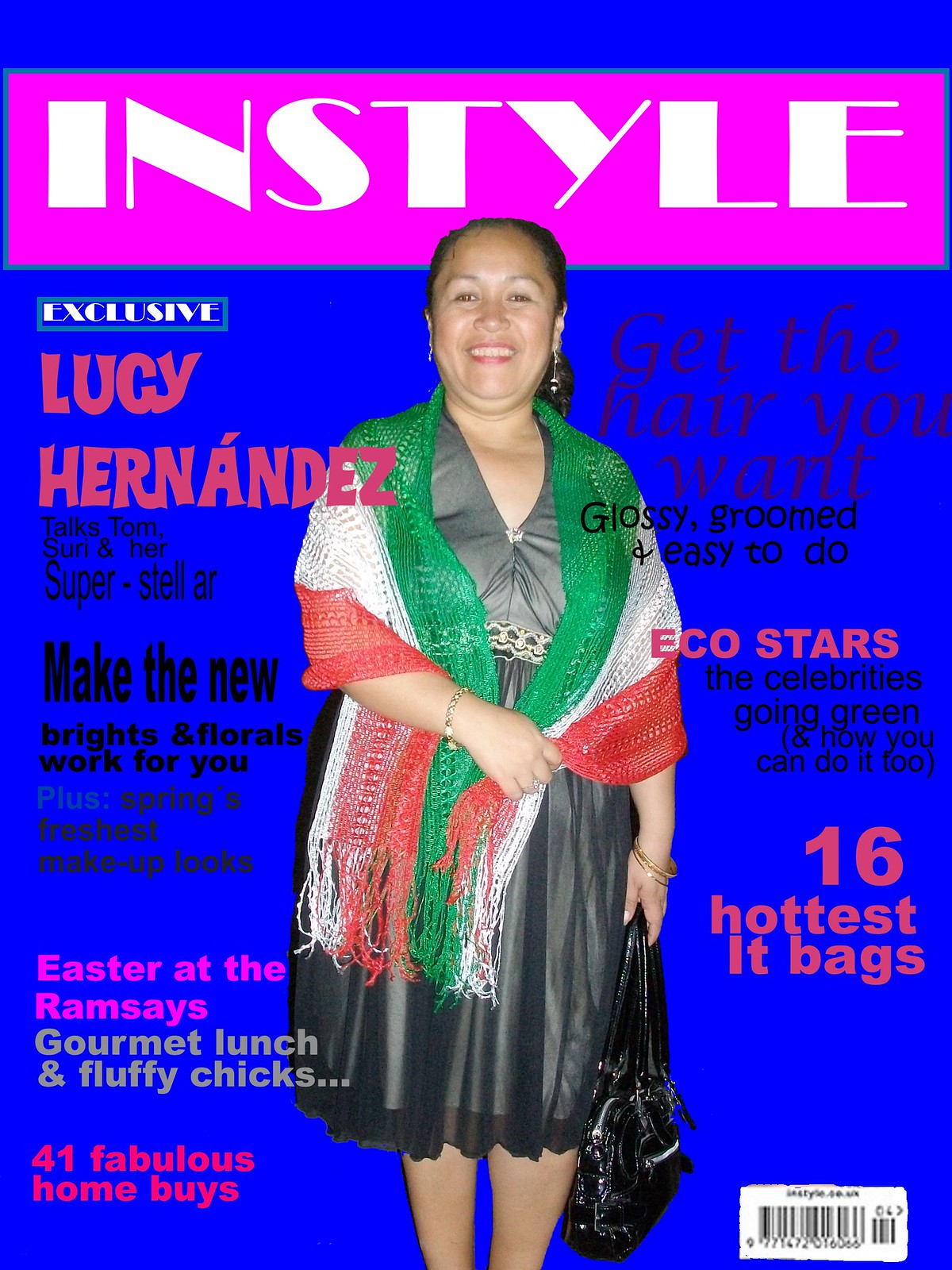The image depicts a digitally-created magazine cover with a vibrant, dark blue background. At the top, a bold pink banner features the title "In Style" in white capital letters. The centerpiece is a photograph of an older woman, likely Hispanic, with her hair tied back and wearing dangly earrings. She is dressed in a gray-green dress, and draped over her shoulders is a red, white, and green knit shawl. She accessorizes with a gold bracelet and holds a black purse. Highlighted in pink is the name Lucy Hernandez, with accompanying black text stating "Talks Tom, Son, and Her Super-Stellar AR." Additional blurbs include "Make the New Brights and Florals Work for You" and "Spring’s Freshest Makeup Looks" on the left. To the right-hand side, captions read, "Get the Hair You Want: Glossy, Groomed, and Easy to Do" and "Eco Stars: The Celebrities Going Green and How You Can Do It Too." Other features include "41 Fabulous Home Buys," "16 Hottest It Bags," and "Easter at the Ramses: Gourmet Lunch and Fluffy Chicks." The bottom right corner shows a white block with a black barcode.